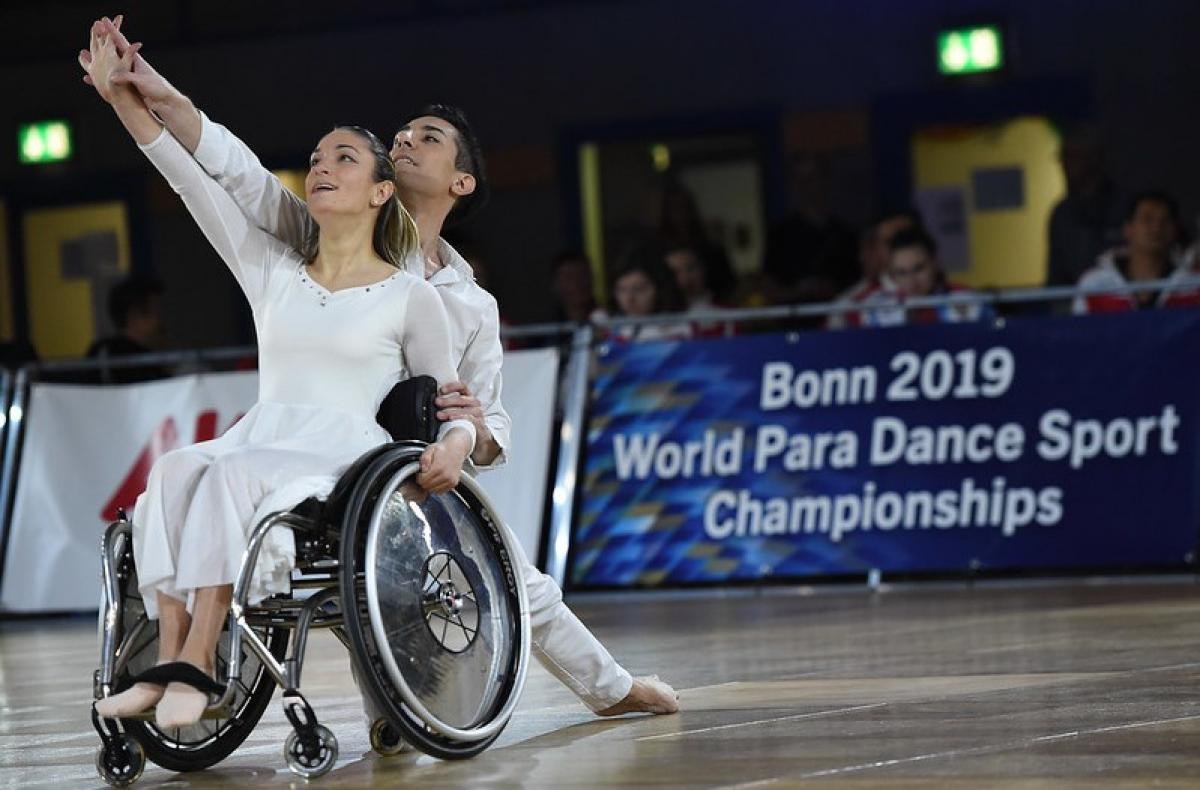In this captivating photograph, taken indoors, the focus is on a woman in a wheelchair and a man behind her, both elegantly dressed in white. The woman, adorned in a long-sleeved white dress with a skirt, has her left hand gripping the wheel of her manual wheelchair for support, while her feet are secured to the chair with black ribbons, possibly to maintain stability. Beside and gently behind her, the man, barefoot and dressed in matching white attire, clasps her right hand as they both extend their arms upwards in a graceful dance pose, looking upwards and smiling. 

In the background, a blue banner with white letters reads "Bonn 2019 World Para Dance Sport Championships," signifying the event. Behind the banner, an audience sits, watching the dancers, their faces out of focus yet displaying expressions of joy and admiration. The backdrop also features hints of yellow and dark colors, creating a contrast that highlights the dancers in the foreground. The image beautifully captures the essence of inclusivity and the elegance of para dance sports.